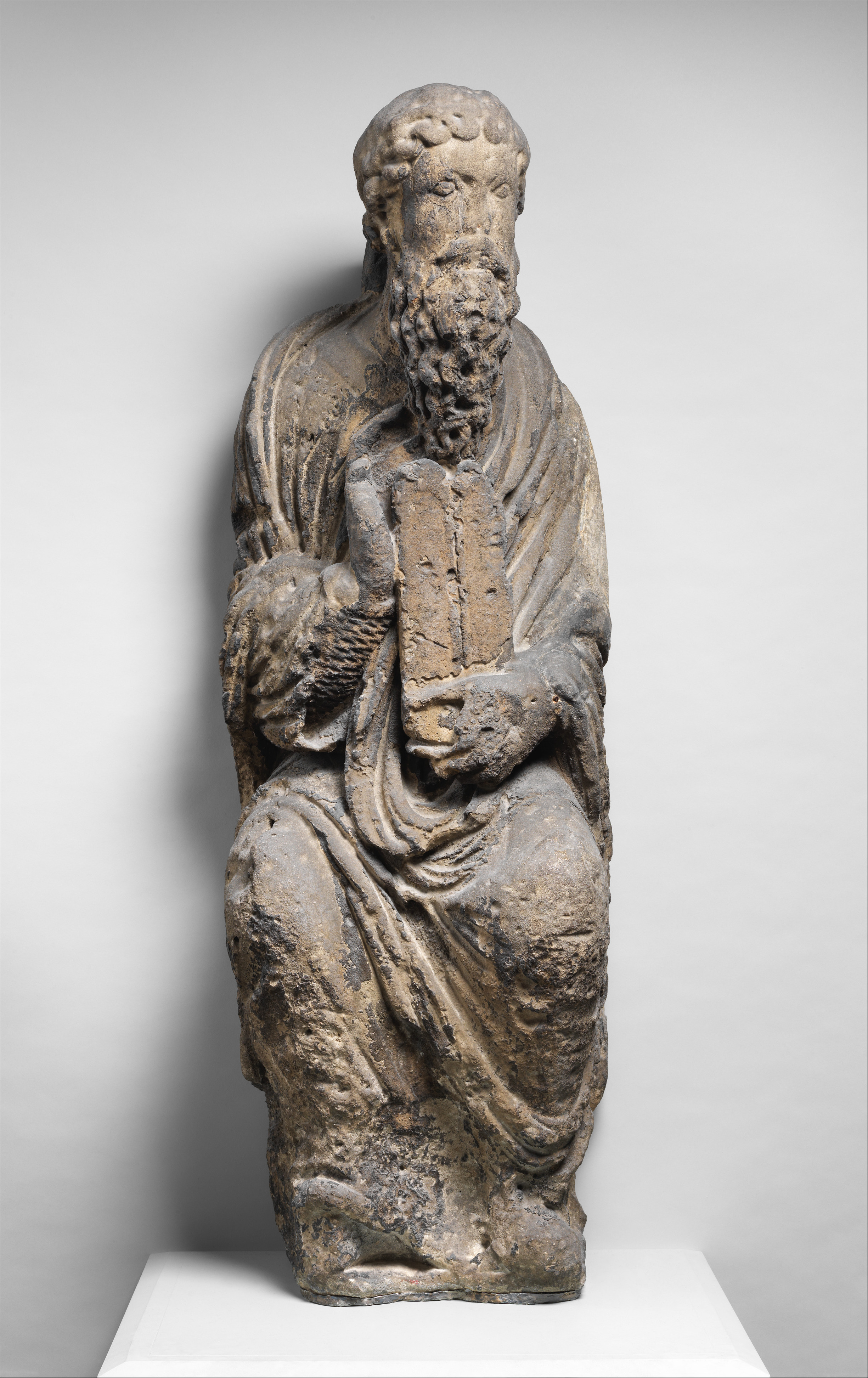The image depicts an aged stone sculpture of an old Greek figure, possibly from Athens. The figure is intricately detailed, showcasing a seated man with a textured beard and curled hair, adorned with a crown of leaves around his head. He wears a meticulously carved robe that drapes between his legs and appears to be holding a scroll or book in his hands. The stone itself exhibits a multi-tonal palette, predominantly featuring grays, with streaks of beige and bronze-like hues, and areas where time has chipped away, revealing white spots of deterioration. The sculpture stands on a white base against a white background, emphasizing its antiquity and the wear it has endured over the years.